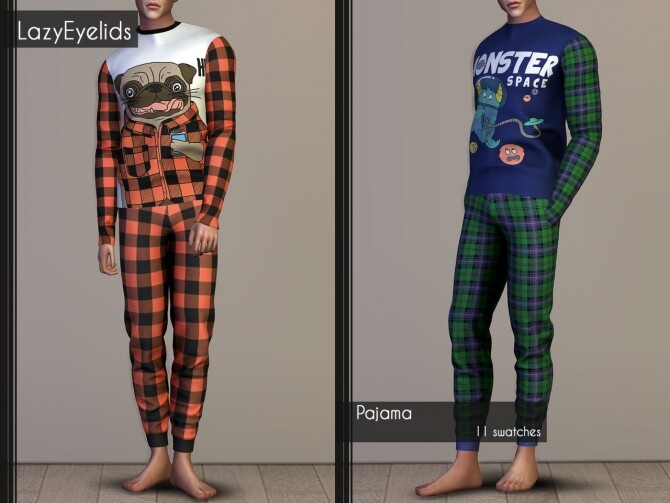The image showcases a split photograph, featuring two computer-generated male models wearing different sets of plaid pajamas, highlighted against a white background. The model on the left is shown from the mouth down. He is dressed in a red and black plaid pajama set with long sleeves and matching pants. His pajama top features a cartoon dog with its tongue hanging out, wearing a matching red and black plaid shirt and holding a phone. The model on the right, similarly depicted from the mouth down, wears green and dark blue plaid pajamas with matching sleeves and pants. His pajama top is dark blue and displays the text "Monster Space" accompanied by a light green cartoon monster with yellow horns and another circular cartoon monster looking frightened. The image includes watermarks reading "Lazy Eyelids" at the top left and "Pajama 11 Swatches" at the center right, suggesting it is an advertisement for pajama designs.